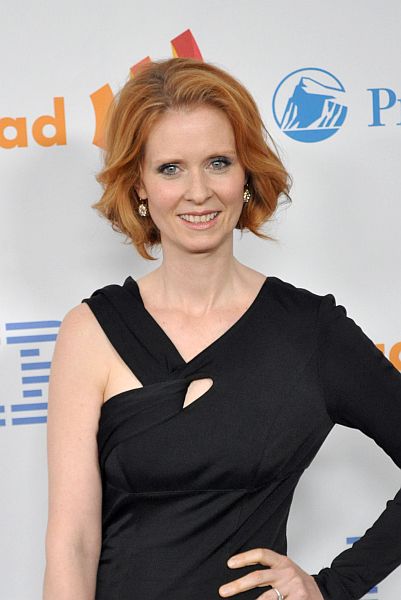In this photograph, actress Cynthia Nixon, known for her role in "Sex and the City," is seen posing at what appears to be an event. The backdrop features a mixture of logos and text, including an IBM logo, an orange logo with signal patterns, and a Prudential insurance blue logo, all printed on a white display board. Cynthia is standing confidently with her left hand on her hip, wearing a unique black dress that has a strap on her right shoulder while the left shoulder is more covered. Her hair is a striking red-orange color, cut short, and she has blue or gray eyes. She accessorizes with dangling silver earrings and a ring on the ring finger of her left hand. Additionally, she's sporting light pink lipstick and soft makeup, completing her elegant look with a gentle smile.